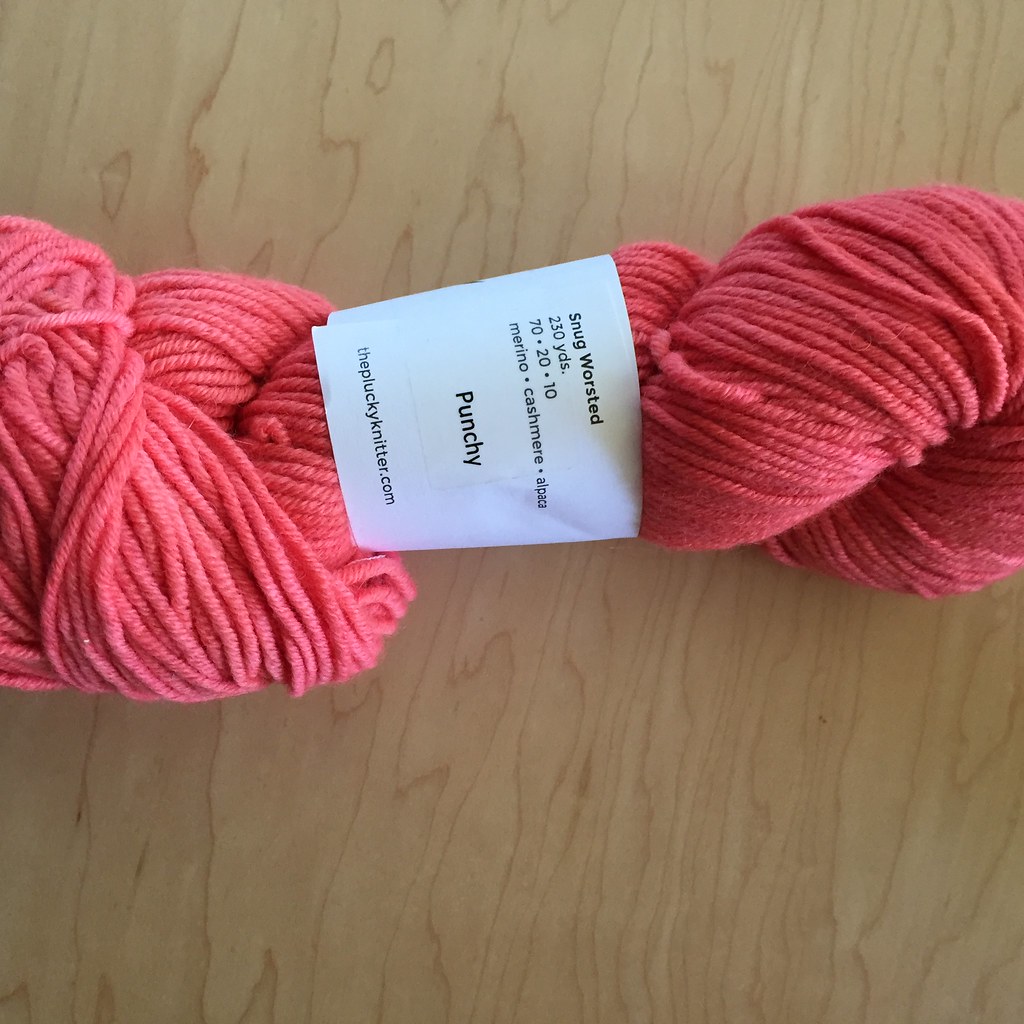The image displays a neatly wound skein of vibrant medium pink yarn, labeled with a white tag in the middle. This tag is adorned with black text indicating key details: "Snug Worsted," "230 yards," "70.20.10," and "Merino Cashmere Alpaca." Notably, it specifies the color as "Punchy" and features the website "thepluckyknitter.com," likely the store from which the yarn originates. The yarn rests on a light brown surface with dark wood grain patterns, suggesting it is placed on a table or desk. The skein is oriented sideways and the picture appears to be taken from a top-down perspective, capturing the detailed text on the tag despite its rotated position. The vivid color of the yarn, reminiscent of a pinkish-red hue, stands out against the subtle wooden background.